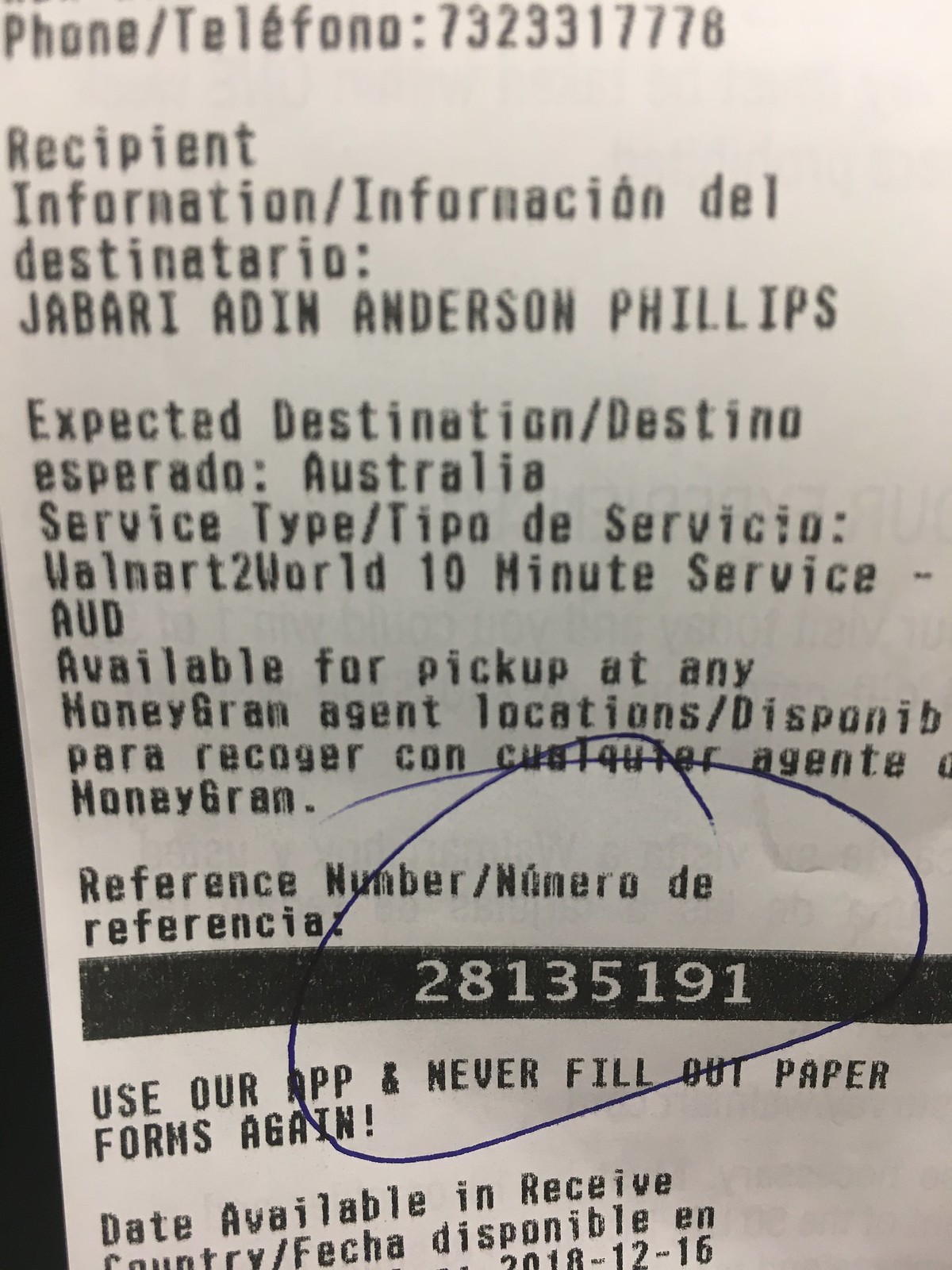This detailed close-up photograph features a white receipt paper, predominantly showcasing a transaction made via MoneyGram. At the very top, the receipt displays a telephone number, 732-331-7778, likely belonging to the business handling the transaction. Directly below, the receipt provides recipient information, identifying the individual as Jabari Adin Anderson Phillips, with an expected destination of Australia, indicating an international money transfer. At the bottom portion of the image, a black stripe contains a series of numbers labeled as the reference number, specifically 281-351-91, which has been circled in blue ink for emphasis.